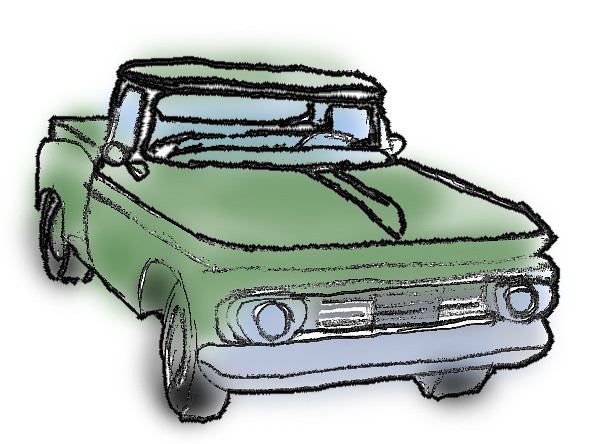The image depicts a detailed, digital rendering of a vintage 1950s or 1960s green Chevy truck, reminiscent of the one driven by Bella Swan in the Twilight movies. The truck is set against a plain white background, with a somewhat messy, sketch-like appearance suggesting it could have been scanned in and then colored using Photoshop. The linework, appearing as though drawn in black ink, exhibits a crayon-like texture. The body of the truck is painted in a splotchy grass green with an airbrushed finish. The tires and the front bumper, along with the grill, are shaded in dark gray, while the interior of the cab and various small accents around the edges of the truck are rendered in a silvery blue and faint purples. The front headlights and the curved edges of the windshield are clearly visible, enhancing its iconic vintage look.